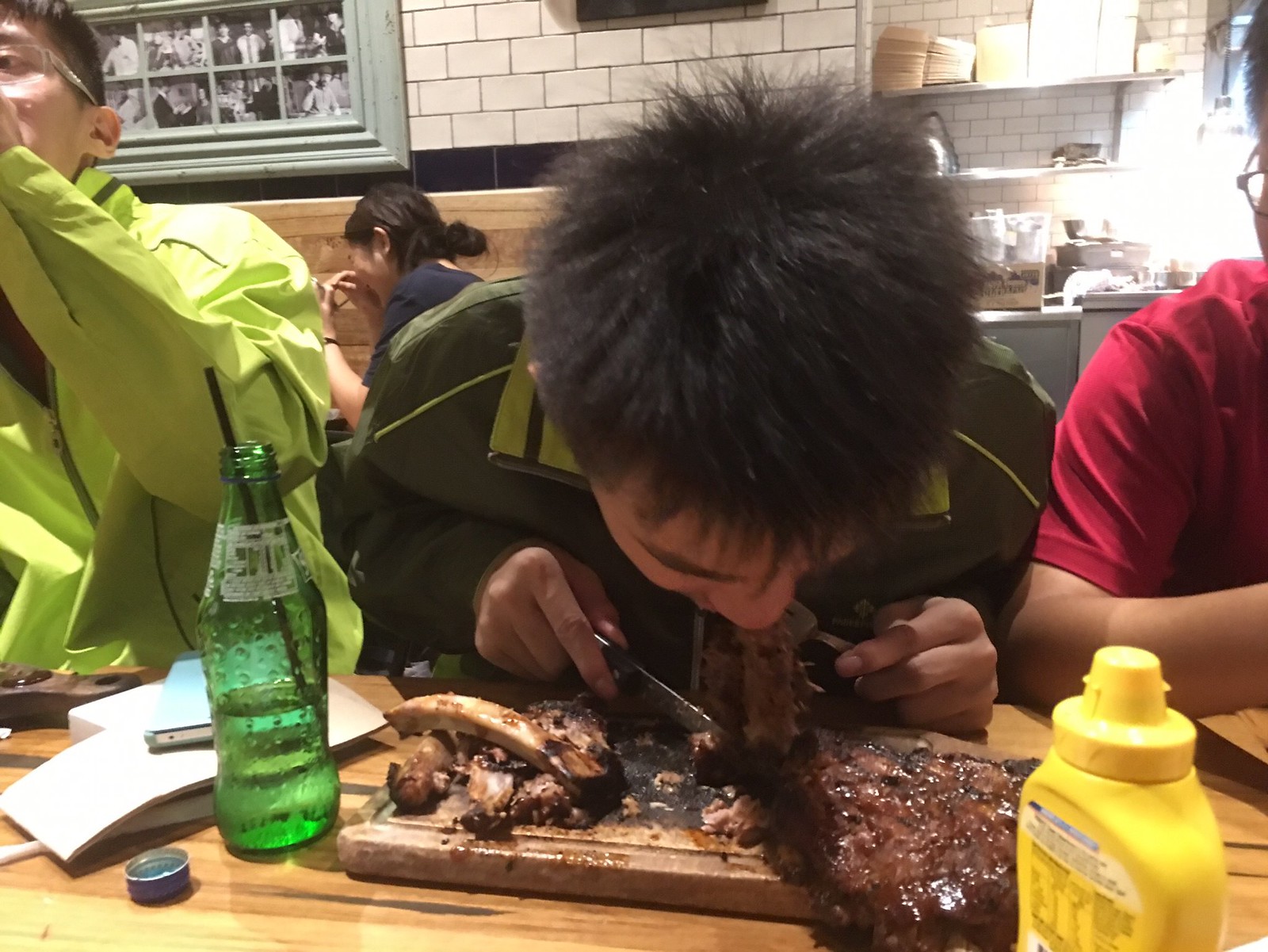In the image, a man, clad in a dark green track jacket with light green trim, is enthusiastically eating a steak on a butcher block-style wooden plate. His head is bent low towards the table, fully immersed in his meal, revealing only the top of his shaggy hair. The steak features bones set aside, indicating he is digging into ribs. In front of him, on the wooden table, there is a bottle of Sprite with a black straw and a bottle of mustard located towards the bottom right corner.

The scene is set against a white subway tile wall with a green-bordered frame displaying a collage of photos. To the man's left, a woman with short, brown hair in a bun, is laughing with her face pointed down, hands pressed together near her face. Further to his left, just partially in the frame, is a man in a bright green jacket. On his right side, partially cut out of the image, is a person in a red t-shirt.

In the background, glimpses of the restaurant kitchen show various boxes, pots, pans, and containers, adding to the bustling atmosphere. There is also a light blue smartphone resting on a stack of papers on the table. This lively scene captures the essence of a busy, convivial dining experience.